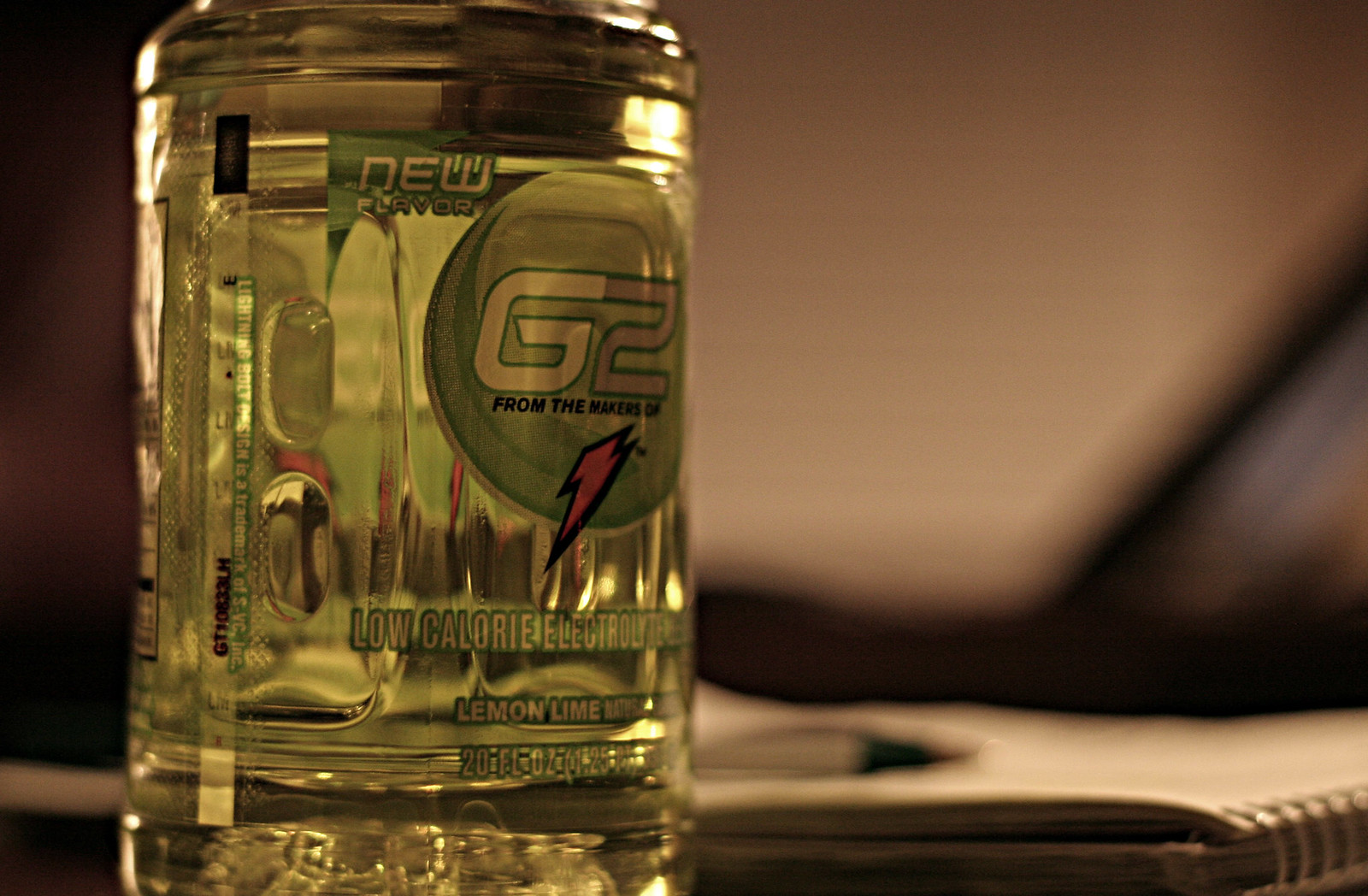This color photograph features a clear plastic bottle of Gatorade filled with a light green liquid. The bottle's label is partially obscured due to the angle, but notable details include the phrase "New Flavor" and a green circle with "G2" in white, indicating it comes from the makers of Gatorade, as symbolized by an orange lightning bolt. The label also reads "Low Calorie Electrolyte Drink, Lemon Lime, 20 Fluid Ounces." The cap is not visible as it is cut off at the top of the image. The bottle is set on a reflective surface, creating a mirrored image beneath it. The background is blurred, keeping the focus on the Gatorade bottle.